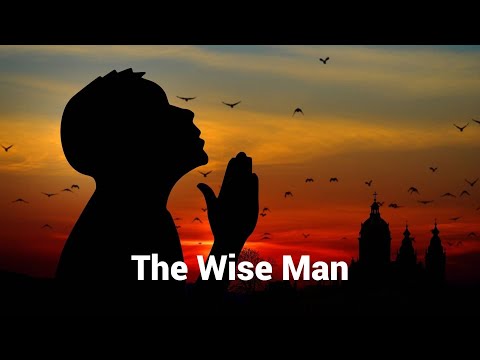In the image, there's a silhouette of a man with his hands raised, seemingly in a praying posture, looking up toward the sky. The man is positioned near the center-left of the image, and his figure is completely black, resembling a shadow. The sky behind him transitions from a deep reddish-orange near the horizon, indicating either a sunset or sunrise, into lighter colors, with a few clouds scattered across. The image also features a flock of black birds flying in the sky, adding to the serene yet mysterious atmosphere. Below the man's silhouette, in a crisp white font, the words "THE WISE MAN" are prominently displayed. The background includes three small buildings with pointed tops or crosses on the right-hand side, suggesting an ancient city skyline. A small tree is also visible in the background. The entire composition is framed by a black border, narrower at the top and wider at the bottom, emphasizing the central elements of the scene. The main colors of the image are the vibrant hues of the sunset or sunrise, contrasted with the stark black of the silhouette and border.